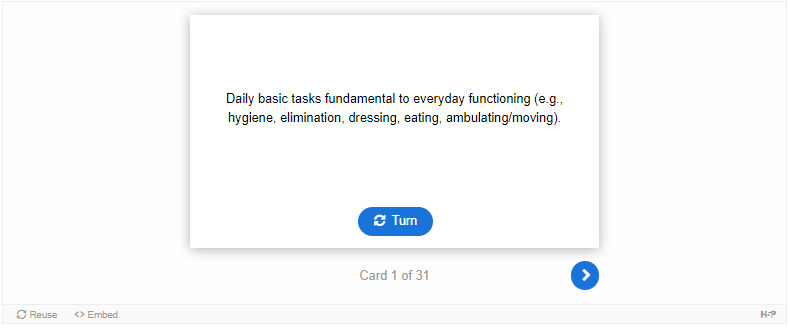The image prominently features a variety of instructional elements overlaid on a website interface designed for flashcards. In the bottom left corner, there is a depiction of an individual named Reeves lying in bed, shown transitioning to a different position, possibly illustrating a task related to personal care or mobility. Adjacent to this, there is a text label that reads "Great Texas card 1 of 31," accompanied by a blue circle and a red arrow for visual emphasis. 

At the center of the image, there is a square shape, distinguished by its tactile black tie design. Below the square, a series of text outlines "Daily basic tasks, fundamental to everyday functioning," specifying activities such as hygiene, elimination, dressing, eating, and ambulating/moving. Parenthetical descriptions further clarify these tasks, giving examples like hygiene and dressing.

Above the central square, there is a blue rectangle labeled "turn," indicating an interactive element, perhaps suggesting that the card can be flipped to reveal additional information.

Subtle shadows are visible along the edges of the image, adding depth and focus to the main elements. The overall interface seems to be from a website dedicated to educational flashcards centered around daily living activities, encouraging users to engage with and learn about fundamental tasks essential for everyday functioning.